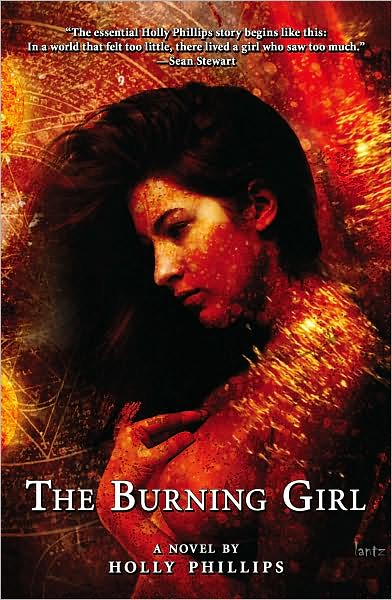The book cover features a central image of a woman, topless and positioned in a side view with her head turned down towards the left. Her long, dark hair cascades over her head and down in front of her body, with one hand delicately placed on her chest, partially covering her breast. The background is a mix of fiery red and orange hues, evocative of flames or possibly fireworks, overlaid with cryptic symbols and what appears to be a partial map or cursive writing that gives an impression of being on fire. Intriguing details like a pentagram near the bottom add to the mysterious vibe. At the very top, in white text, a book review reads: "The essential Holly Phillips story begins like this: In a world that felt too little, there lived a girl who saw too much. – Sean Stewart." At the bottom of the cover, the title and author are prominently displayed: "The Burning Girl, a novel by Holly Phillips." The overall effect is one of intrigue and dark allure, drawing the viewer into the enigmatic story within.